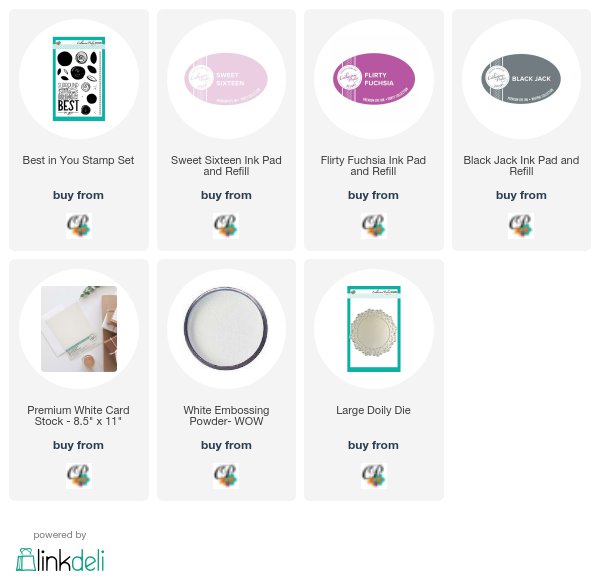The image appears to be a screenshot from a website dedicated to stamp and crafting supplies. At the top, there are four distinct rectangular sections:

1. **Top Left Rectangle**: Labeled “Best in Use Stamp Set,” it includes a clickable link indicated by a thumbnail of the brand’s logo.
2. **Second Rectangle**: Titled “Sweet 16 Ink Pad and Refill,” it mirrors the layout of the first with a thumbnail logo for purchasing.
3. **Third Rectangle**: Featured as “Flirty Fuchsia Ink Pad and Refill,” again with a clickable logo for buying.
4. **Fourth Rectangle**: Named “Blackjack Ink Pad and Refill,” also includes a clickable logo for purchasing.

In these sections, there are images representing the respective stamp sets and ink pads.

The lower row comprises three additional rectangles:

1. **Bottom Left Rectangle**: Highlights “Premium White Card Stock 8.5" x 11"” with an accompanying image of the card stock.
2. **Middle Rectangle**: Describes “White Embossing Powder W.O.W.” and similarly includes a clickable logo for buying.
3. **Rightmost Rectangle**: Labeled “Large Doily Die” with an image of the doily and a clickable logo.

In the bottom left corner of the screenshot, there is a label that reads “Powered by Link Deli,” accompanied by a graphic of a shopping bag preceding the word "Link." 

Overall, the layout is visually organized to highlight various stamping and crafting products, complete with convenient purchase links.